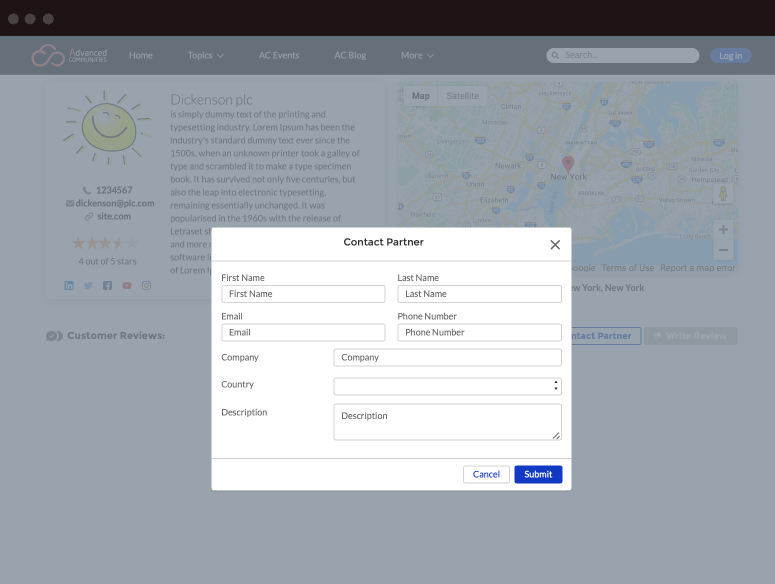The image features a website with a predominantly pink theme. On the left side of the screen, there is a pink symbol and a navigation menu that includes options such as Home, Topics, AC Events, AC Blog, and more. The background also displays an icon of a sunshine, drawn in a childlike manner, adding a playful touch to the design.

Underneath this navigation menu, there is a detailed section for customer reviews, showcasing a rating of four out of five stars. The reviews are hosted on a website named Dickinson-something.com, specifically under a section titled "Dickinson Pics" or "Pictures". The site features classic placeholder text, often known as "Lorem Ipsum." The text is an industry-standard used in printing and typesetting since the 1500s, when it was first used by an unknown printer to create a type specimen book. This text has remained largely unchanged and continues to be a staple in electronic typesetting today.

In the foreground, there is a pop-up contact form titled "Contact Partner." The form requests users to input their first name, last name, email, phone number, company name, and country (selectable from a drop-down menu). Additionally, there is a field for a brief description of the user. After filling out the required information, users can choose to either cancel or submit the form by clicking a blue button.